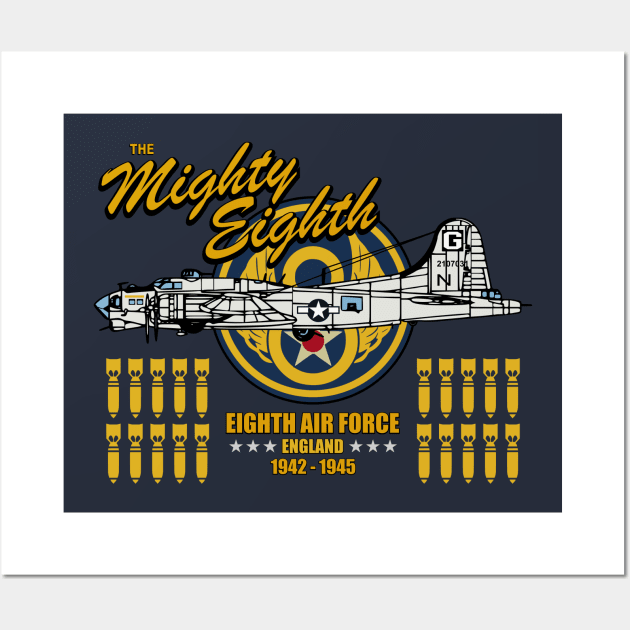This is an image of a poster for the Mighty Eighth Air Force, active from 1942 to 1945 in England. The poster has a dark gray background with a white border. At the top left, in yellow cursive font, it reads "The Mighty Eight." Below, there is a white World War II bomber aircraft depicted in profile, with a US Army Air Corps star featuring a blue circle. On the wing, the aircraft has markings including the letter "G" and the numbers "2107031," with an additional "N" noted below. Behind the aircraft is the emblem of the Mighty Eighth, a yellow circle with a red-centered star and wings extending from each side. In the middle third of the image, it states "Eighth Air Force, England, 1942-1945," flanked by two rows of five bombs on each side. The detailed artwork and emblem reflect the historical significance of the Mighty Eighth Air Force during World War II.